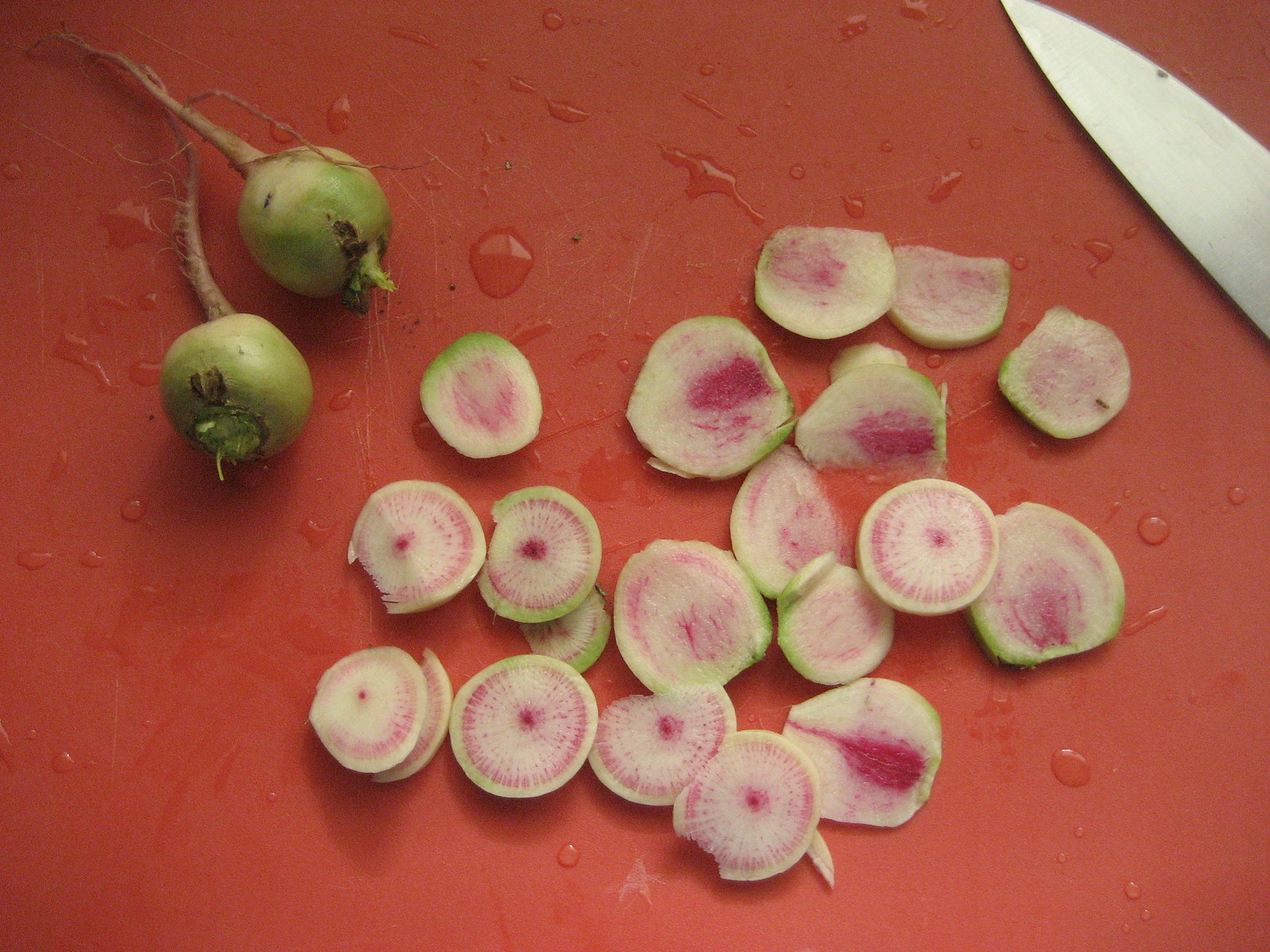This is a detailed overhead photograph of a vegetable, likely a radish, on a red cutting board with visible scratches. The image captures a scene where this vegetable has been sliced into circular pieces. The radial slices feature a green outer layer with a red interior and white outlines, creating a starburst effect transitioning from dark red in the middle to lighter shades toward the edges in an ombre pattern. Water droplets are scattered across the slices, indicating the vegetable was wet when cut. In the upper left corner are two whole radishes, distinguishable by their green bodies and brown roots. In the top right corner, a silver knife rests, suggesting it was used for slicing. At the bottom of the image, a white letter 'A' is visible, adding a distinct element to the composition.